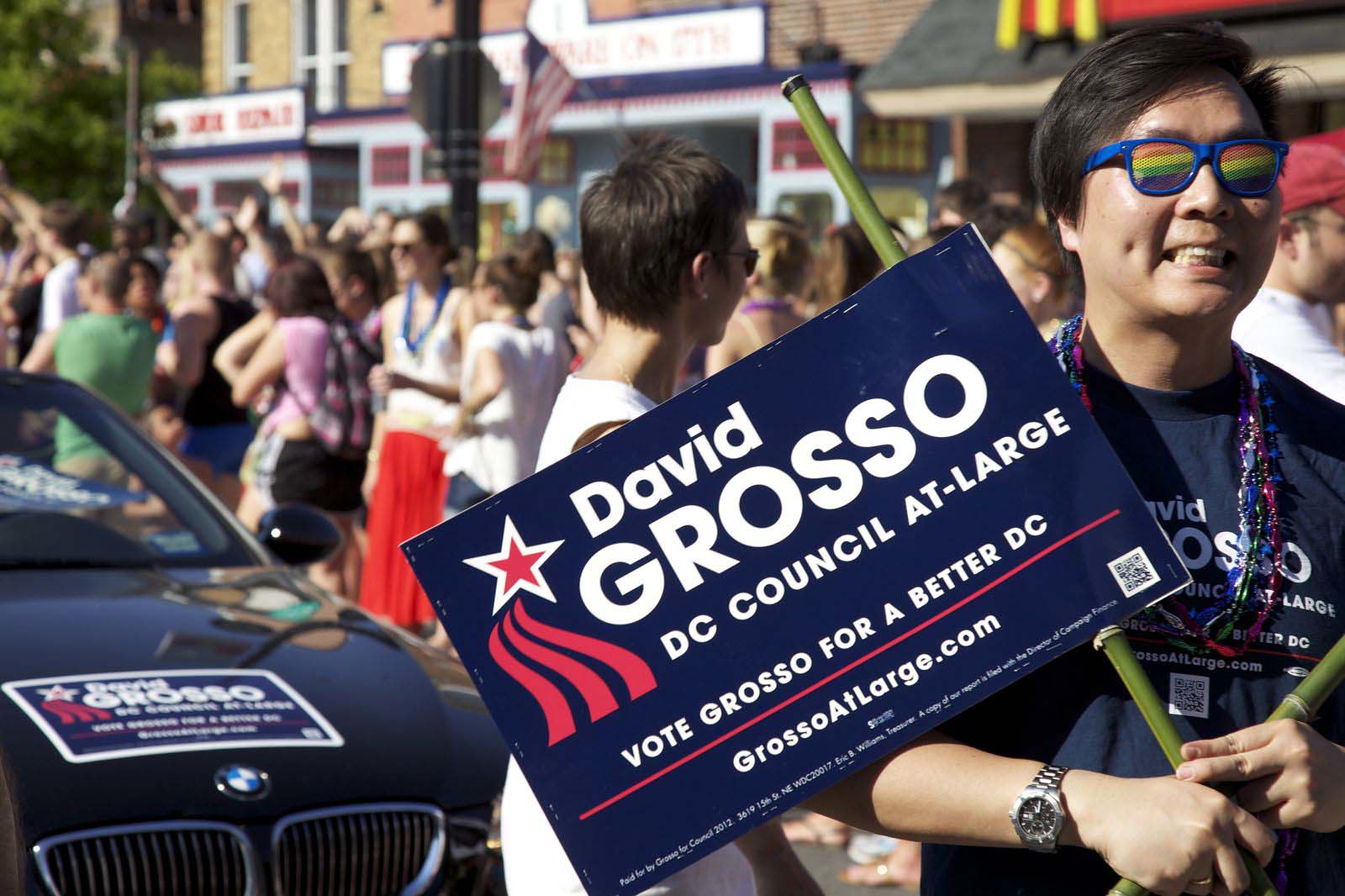In the image, a vibrant political rally unfolds on a sunny day. At the forefront, an Asian man wearing rainbow sunglasses and a blue t-shirt emblazoned with "David Grosso" holds a prominent navy-blue banner on a green pole. The flag, featuring a red star and wavy white stripes, reads "David Grosso, D.C. Council-at-Large" and "Grosso-at-Large.com." He sports a watch on his left wrist. Behind him, a black BMW also displays a similar campaign sign. The rally scene is bustling with numerous people and is set against an urban backdrop that includes visible buildings, a McDonald's restaurant, and green trees. An American flag is noticeably present, contributing to the patriotic atmosphere of the event.